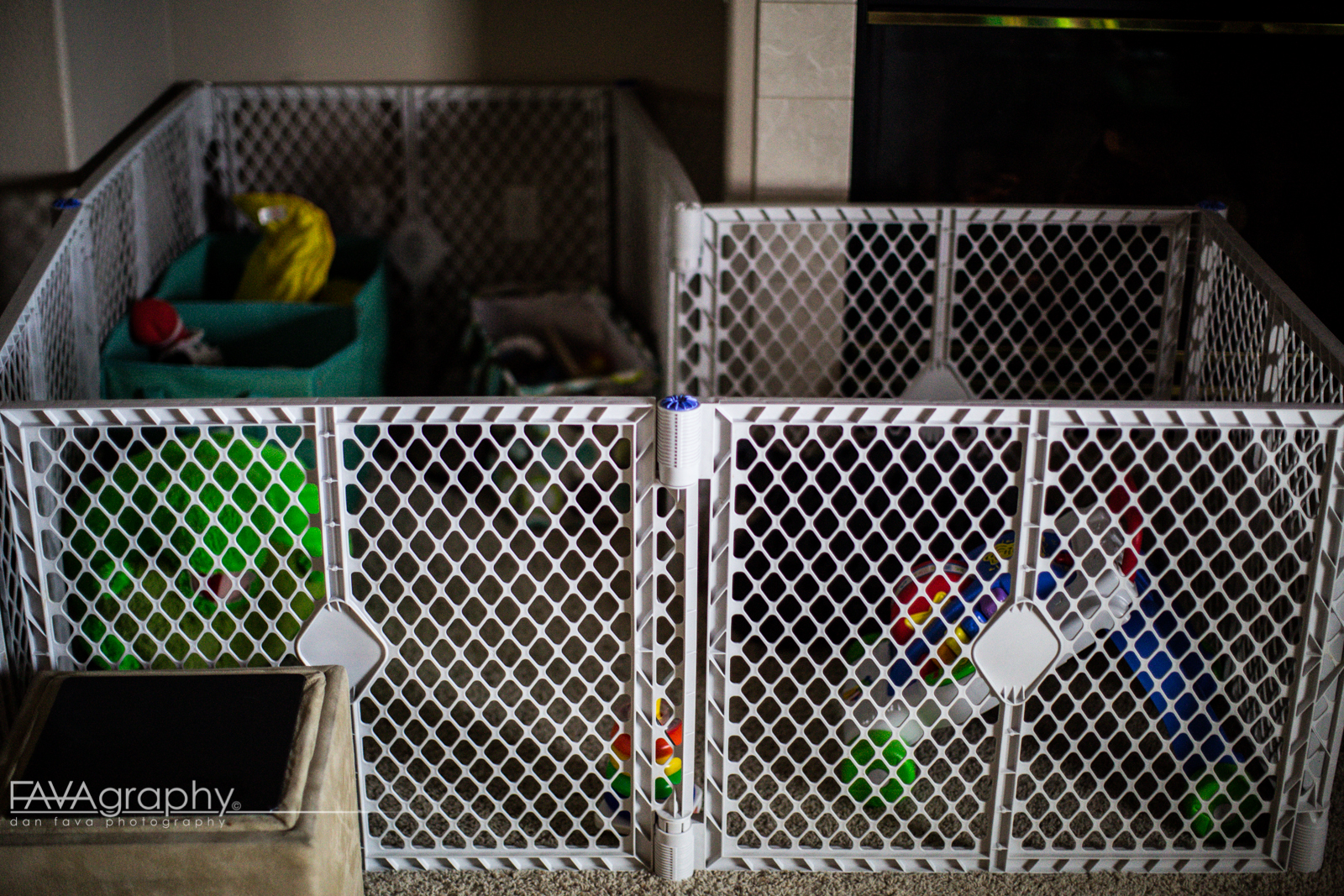This detailed color photograph depicts a grey plastic L-shaped enclosure, resembling a playpen commonly used for puppies or children. The playpen, set up in what appears to be a dimly lit garage, is constructed from several panels featuring triangular mesh-like openings. Inside the enclosure, an assortment of children's toys is visible. Among the toys, there is a brightly colored plastic activity center on one side, which includes front wheels and a balancing pole at the back. Near it, a classic Fisher-Price stacking ring toy stands out. Alongside these, there are two toy storage bags: a smaller, longer one and a green bag divided into two pouches, both brimming with toys. On the bottom left side of the photograph, the words "Fava Graphy, Don Fava Photography" are inscribed. Also present in the foreground is a small, tan and brown rectangular box.